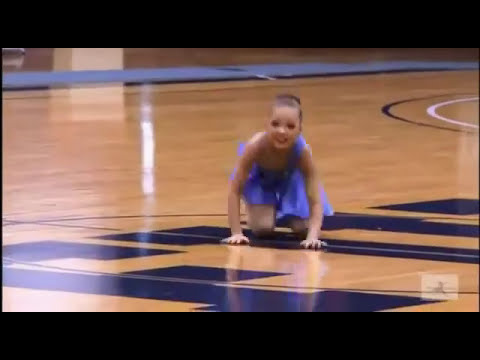The image depicts a young girl, around 10 years old, on an indoor basketball court with a shiny brown hardwood floor, featuring a prominent logo in the center, likely representing the host team or mascot in navy blue. The girl is wearing a light lavender or purple dress resembling a dancer's costume with one strap on the left shoulder and her hair styled in a bun. She appears to be in a crawling position on her hands and knees, with a look of panic or struggle on her face. Surrounding her on the court are various markings and curved blue and white lines. There's a discernible ball-like figure or logo in the bottom right corner. In the background, padded mats line the sidelines, and an off-white pillar is visible. The image, taken in landscape orientation, hints at a large light source on the left, suggesting it might have been captured during a dance routine or some form of contemporary performance.